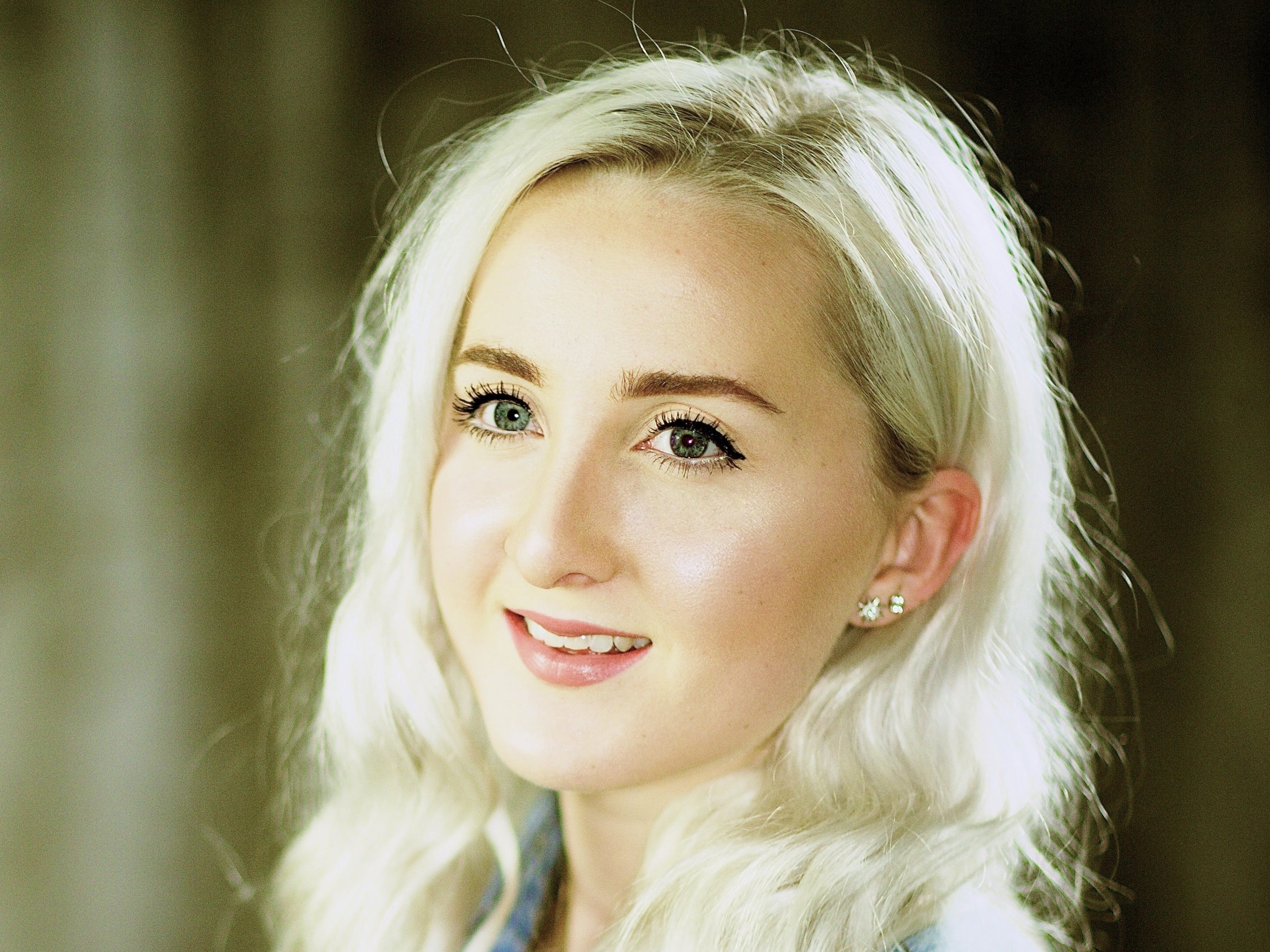The image showcases a professional model photo of a young woman with light platinum blonde hair, visibly dyed with dark roots peeking through. She has striking blue eyes, accentuated with full makeup that includes brown eyebrows, false eyelashes, eyeshadow, eyeliner, and lipstick. She smiles gently, revealing perfect white teeth, and her clear skin glows under bright lighting. In her left ear, which is the side visible in the photo, she wears two earrings. The background is a blurred, green hue that contrasts with her presumed blue blouse, although it's somewhat fuzzy. The overall composition focuses on her head, bringing attention to her facial features and expression.